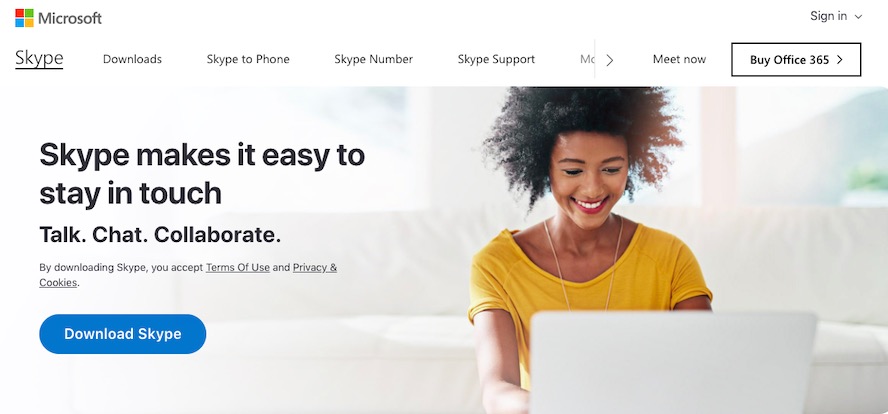A screenshot of a Microsoft web page showcases multiple features related to Skype and Office 365. The web page header displays "Microsoft" in the upper left corner and a "Sign In" option in the upper right. Below the header is a horizontal menu bar listing "Skype downloads," "Skype to phone," "Skype number," "Skype support," "Mic" (partially cut off), "Meet Now," and a boxed option for "Buy Office 365," each accompanied by navigational arrows.

Centrally featured is a vibrant and engaging promotional image. A smiling woman with wild, curly hair that might suggest a mixed-race background is the focal point. She is dressed in a mustard-colored shirt and wears striking red lipstick. She is visibly happy and is working on a white laptop situated on a white table. The image has a minimalist background: a white couch, a window revealing a slice of sky, and subtle interior elements.

Superimposed over the image in bold, large font, the text proclaims, "Skype makes it easy to stay in touch." This is followed by smaller print, emphasizing the words: "Talk. Chat. Collaborate." Lastly, in fine print, the message informs users: "By downloading Skype, you accept Terms of Use and Privacy and Cookies," with "Terms of Use" and "Privacy and Cookies" underlined for emphasis. Below this text, a prominent blue button invites users to "Download Skype."

The overall design of the web page is clean and straightforward, effectively encouraging users to leverage Skype for communication.